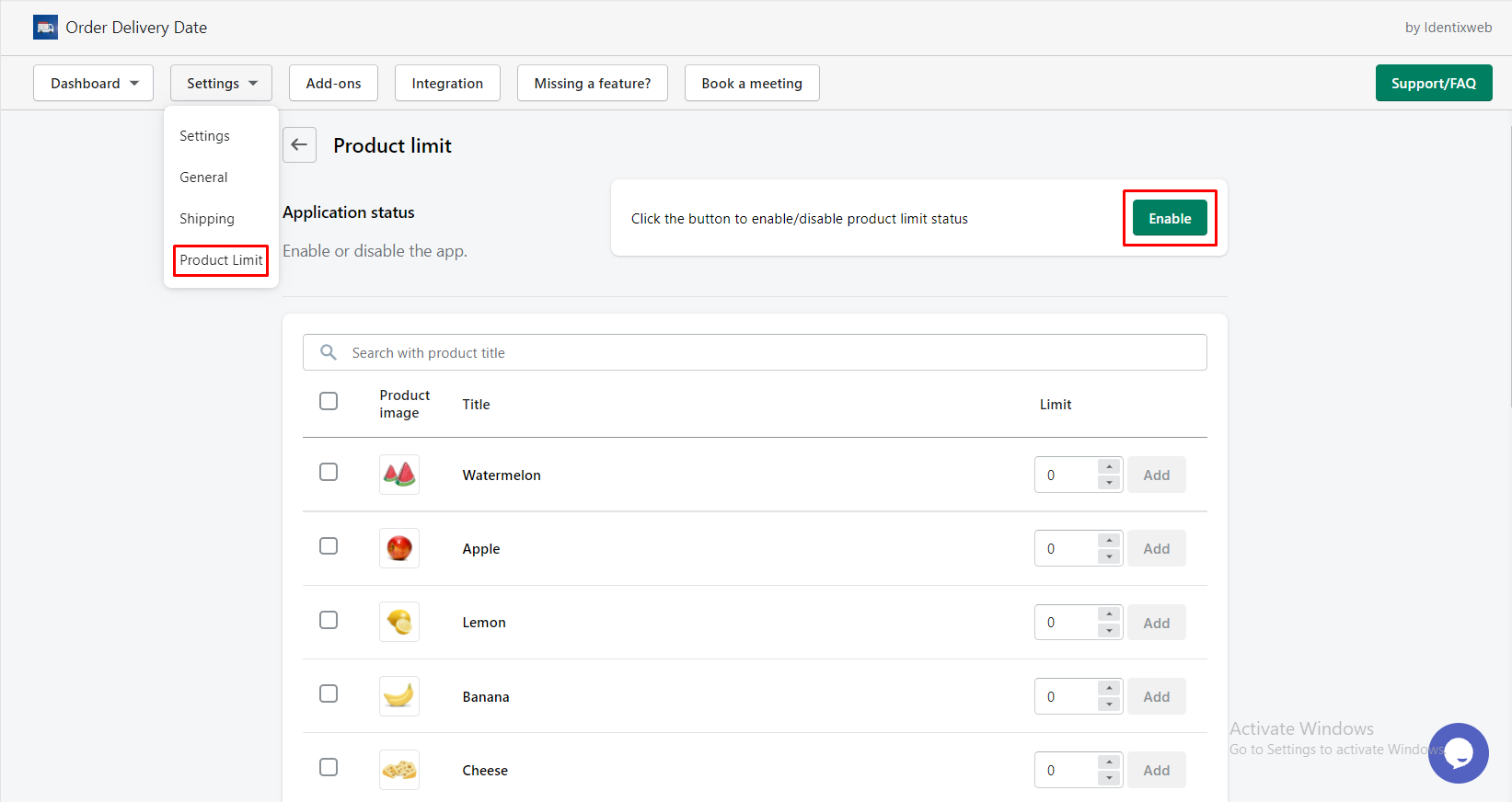This is a comprehensive product ordering interface. 

In the upper left corner, there is a label for "Order Delivery Date." Directly beneath this, a drop-down menu labeled "Dashboard" is available. Following this, another drop-down menu offers various settings options listed as "Settings," "General," "Shipping," and "Product Limit," with "Product Limit" highlighted in red.

Next to these options are additional tabs labeled: "Add-Ons," "Integration," "Missing a Feature," and "Book a Meeting." On the far right, a green rectangle contains the "Support/FAQ" button.

Below these options, the interface displays "Application Status" with an option to enable or disable the app. This feature is controlled by a button labeled "Enable" within a green box, bordered in red.

Underneath the application status, there is a search bar with the placeholder text "Search with product title." Below the search bar, a table is presented which begins with an empty checkbox, followed by columns for "Product Image," "Title," and "Limit."

The first row in the table contains:
- A blank square checkbox
- An image of watermelon slices
- The word "Watermelon"
- The limit set to "0"

The second row contains:
- A blank square checkbox
- An image of an apple
- The word "Apple"
- The limit set to "0"

The third row contains:
- A blank square checkbox
- An image of lemons
- The word "Lemon"
- The limit set to "0"

The fourth row contains:
- A blank square checkbox
- An image of a banana
- The word "Banana"
- The limit set to "0"

The fifth row contains:
- A blank square checkbox
- An image showing pieces of cheese
- The word "Cheese"
- The limit set to "0"